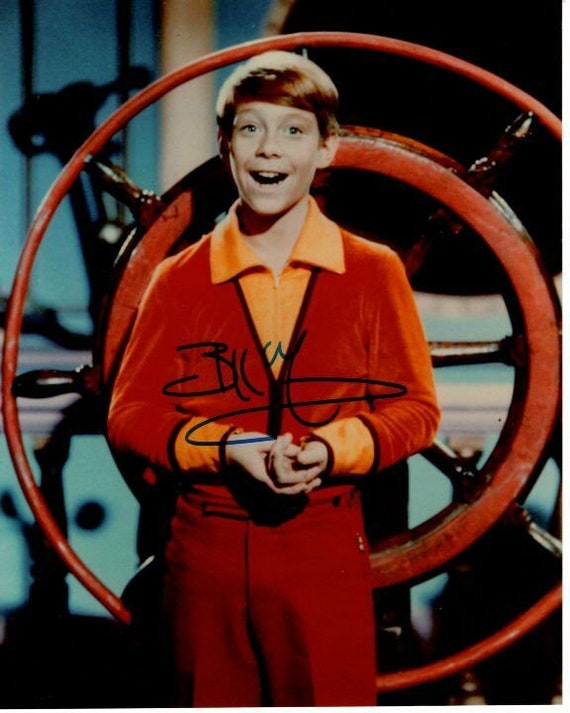A vertically oriented photograph captures a young adolescent boy, approximately 12 or 13 years old, standing confidently in a vivid red and orange sweatsuit. The ensemble comprises a striking red-and-orange top paired with matching orange-red slacks. The boy, who is Caucasian with a head of vibrant red hair, has his hands clasped together at his midsection. His mouth is open, as if caught mid-song, giving the impression that he is singing. The photograph bears the boy’s autograph, adding a personal touch to the image.

In the background is a large, reddish-orange ship's wheel, reminiscent of those used to steer old-fashioned boats. The wheel is held together by wooden spokes positioned between its inner and outer circles. The backdrop further includes indistinct blue-tinted areas and regions of deep shadow, providing contrast that highlights the vibrant colors of the boy’s outfit and the ship's wheel.